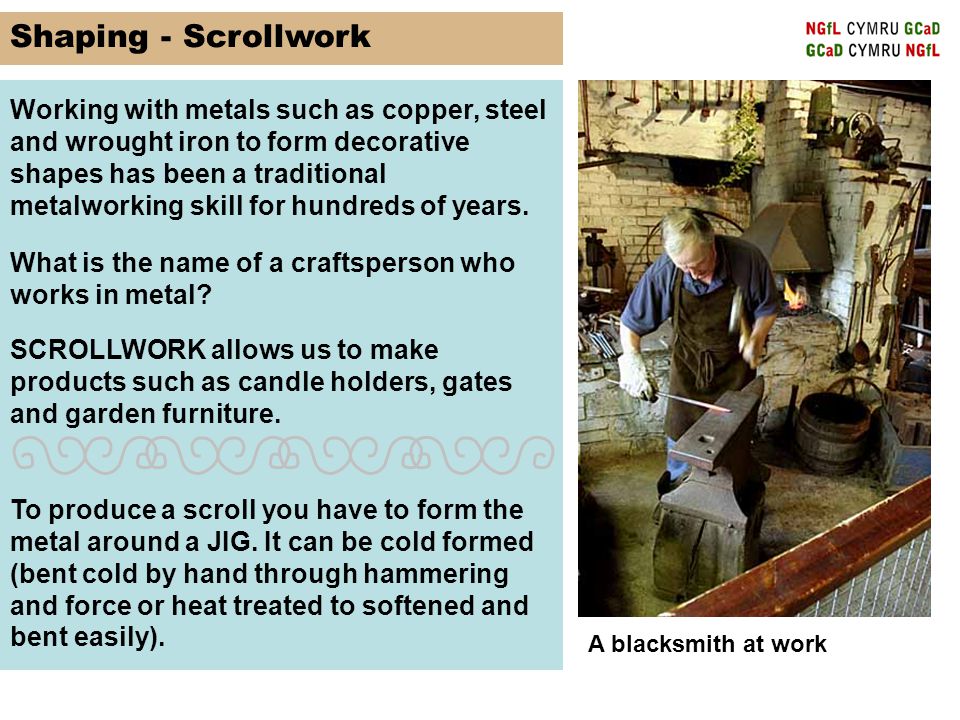The image features an educational slide on “Shaping Scroll Work,” set against a golden background with bold black text highlighting the title. The informative text explains the traditional metalworking technique of shaping metals like copper, steel, and wrought iron into decorative shapes, a skill practiced for centuries. It introduces the craftsperson known as a blacksmith and details the process of scroll work, which allows the creation of items such as candle holders, gates, and garden furniture. The text explains that to produce a scroll, metal must be formed around a jig, either cold by hand using hammering and force or by heat treating to bend easily. Dominating the right side of the image, a photograph captures a blacksmith at work. The blacksmith, wearing a blue shirt and black apron, is in mid-action at his anvil, hammer poised to strike a heated, glowing piece of metal held in his gloved hand. Surrounding him are various tools, a bucket, and a rail, indicating a typical blacksmithing setting. The caption under the picture succinctly reads, "A blacksmith at work," further emphasizing the educational purpose of the image.